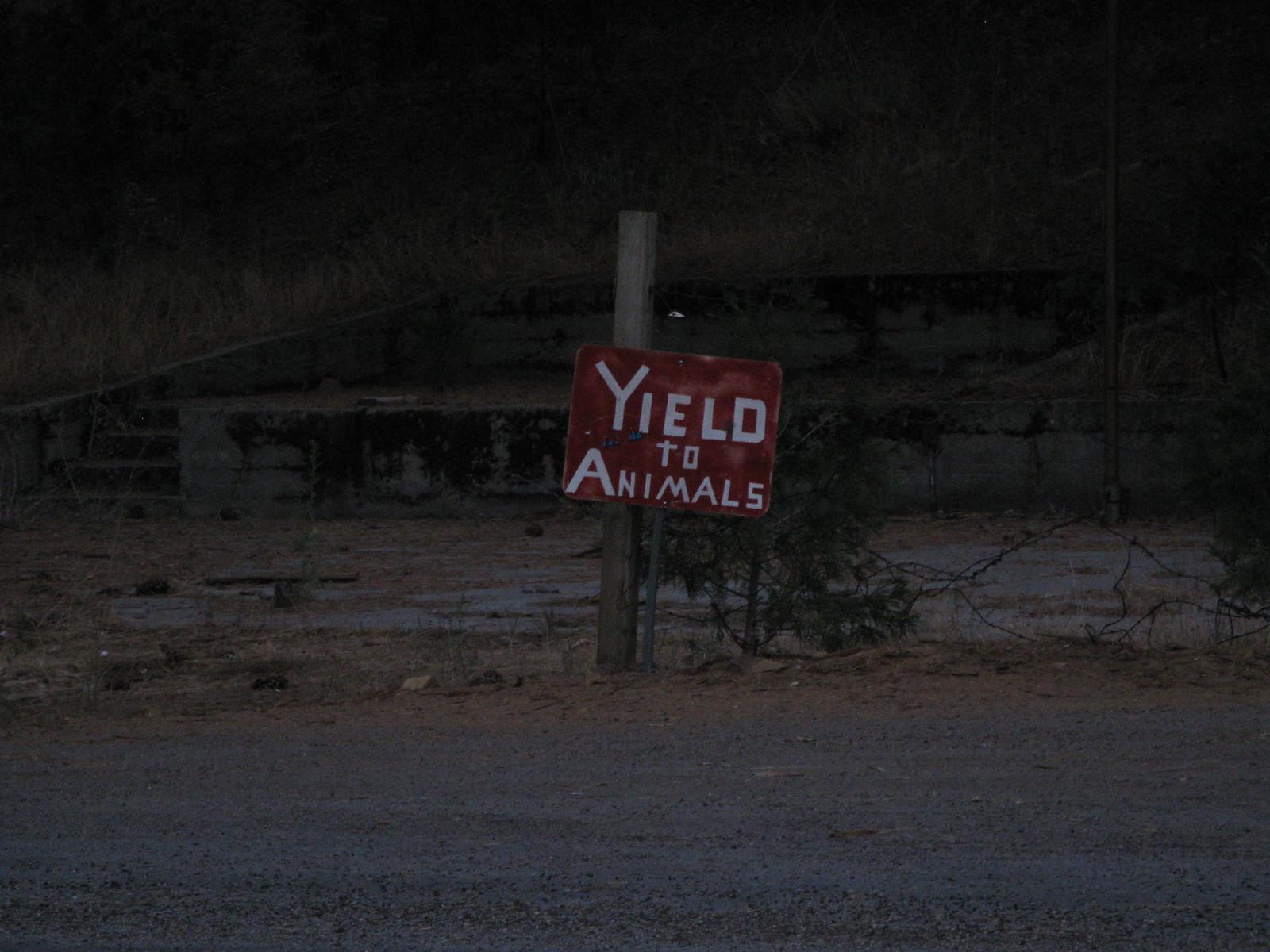This nighttime roadside photograph captures a rugged scene dominated by a red metal sign with white lettering that says "yield to animals," attached to a thin gray pole. The somewhat neglected road in the foreground is gravelly, with dirt and scattered materials, indicating it may not be well-maintained. Around the sign, a mix of dead and green branches, brown grass, and dirt are visible, lending an overall rustic feel. To the side of the sign, a wooden log or stake is noticeable amidst the foliage. In the dimly lit background, a concrete section with three steps leads to a flat, narrow platform, possibly the remains of a small building, highlighted by a low gray brick wall with faded black paint. Further behind, the silhouette of a hill or mountain is faintly outlined against a backdrop of yellow and brown grass. Two small blue stickers are also present near the letters "Y" and "I" on the sign, adding subtle details to this largely monochromatic scene.